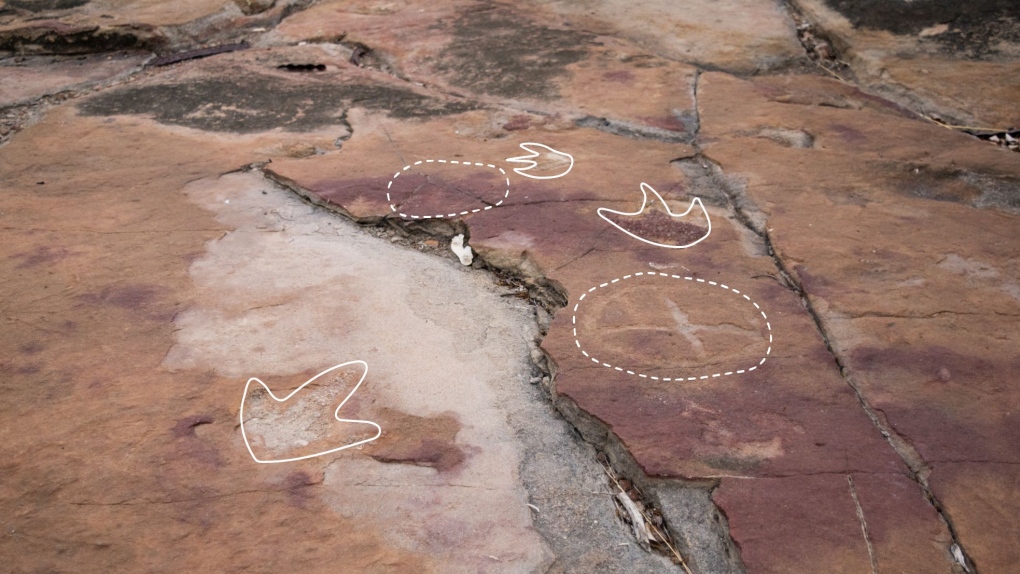This aerial, angled color photograph appears to capture a textured surface that resembles rock or concrete, exhibiting a striking mosaic of multiple tones, including orangey-tan, reddish, and burgundy areas, with touches of green vegetation and white patches. The surface is intricately cracked, revealing gray beneath the fissures, lending a clay-like appearance. Superimposed on this textured canvas are various markings in white: three arrows pointing in different directions, two circular shapes with dotted lines and white Xs at their centers. These annotations seem to highlight specific features, potentially suggesting the presence of fossils within the rock. The combination of natural colors and added diagrams creates a rich, detailed tableau that invites further exploration and interpretation.